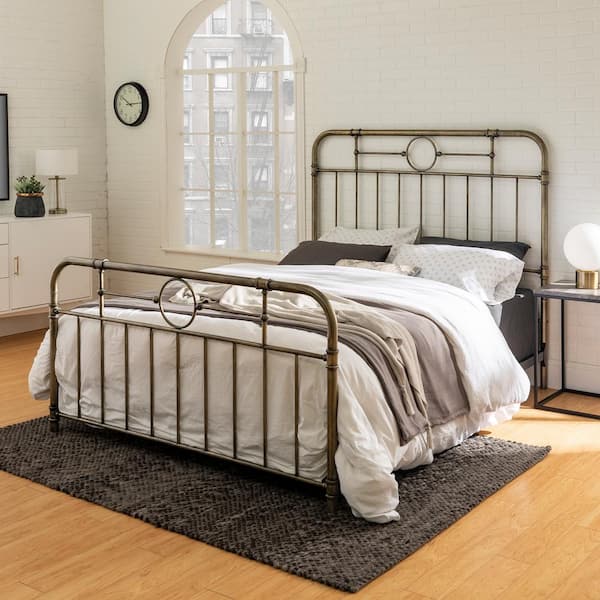This image captures a neat, aesthetically clean bedroom with striking details. The bed, which is the focal point, features a metal frame with a taller headboard and a shorter footboard, both adorned with circular designs and bars. It is made up with a thick white comforter, multiple pillows (gray and white polka dot and solid gray), and a gray blanket at the center. Draped over the foot of the bed is a robe, adding a touch of casual elegance. The bed rests partially on a large gray rug that contrasts against the light wooden floor.

To the right of the bed, there is a mostly-wire nightstand topped with a globe-like white lamp resembling a crystal ball. To the left, an arched window covered with bars is a distinctive architectural feature. Adjacent to it, you can see a white dresser with gold handles, which supports a black potted plant and a white lamp. On the wall above, there's a hint of a black television, and in the left corner, an old-time analog clock adds a touch of vintage charm. The bedroom's walls appear to be white brick, enhancing the room's sparse, yet cozy aesthetic.